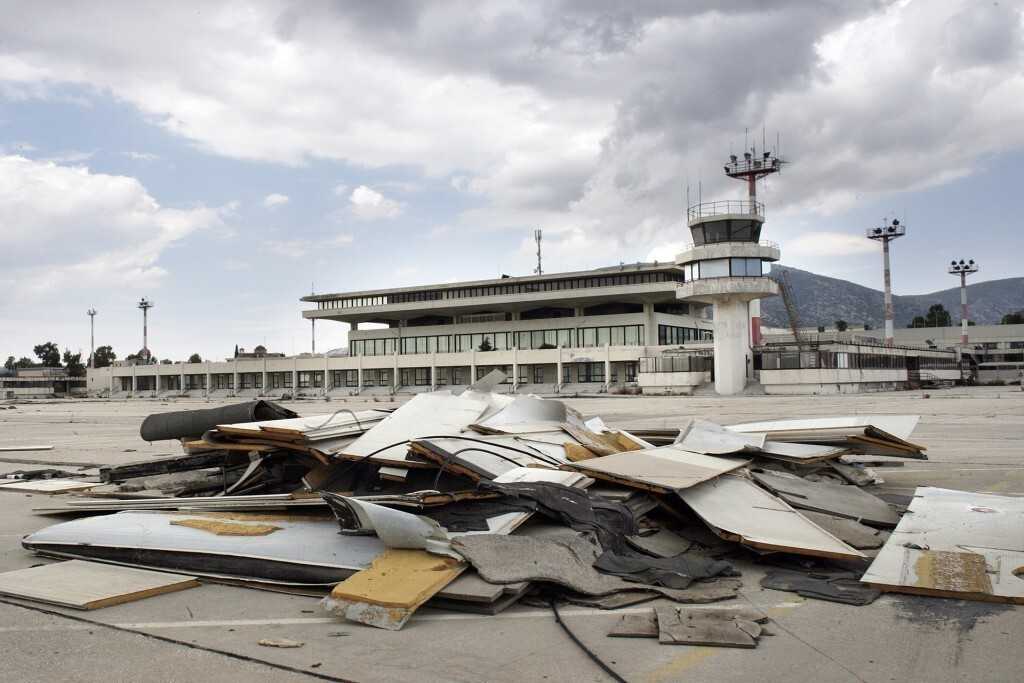The photograph captures a gloomy, overcast day at what appears to be an abandoned airport. The foreground is dominated by a substantial heap of debris scattered across the tarmac, including metal and wooden panels, insulation, carpet remnants, and other construction materials. This pile likely results from a demolished building, given its composition resembles office ceiling tiles or floor panels. The background features a large, two-story terminal building characterized by extensive glass-front windows and a central antenna atop its roof. To the right of the terminal is a prominent, shorter, round tower with a black, octagonal observation area encircled by railings. Further in the distance, multiple utility towers align sequentially, both to the right and left of the terminal. The entire scene is underscored by a fence stretching across the view, with dark, foreboding clouds filling the sky above, casting a somber mood over the area.